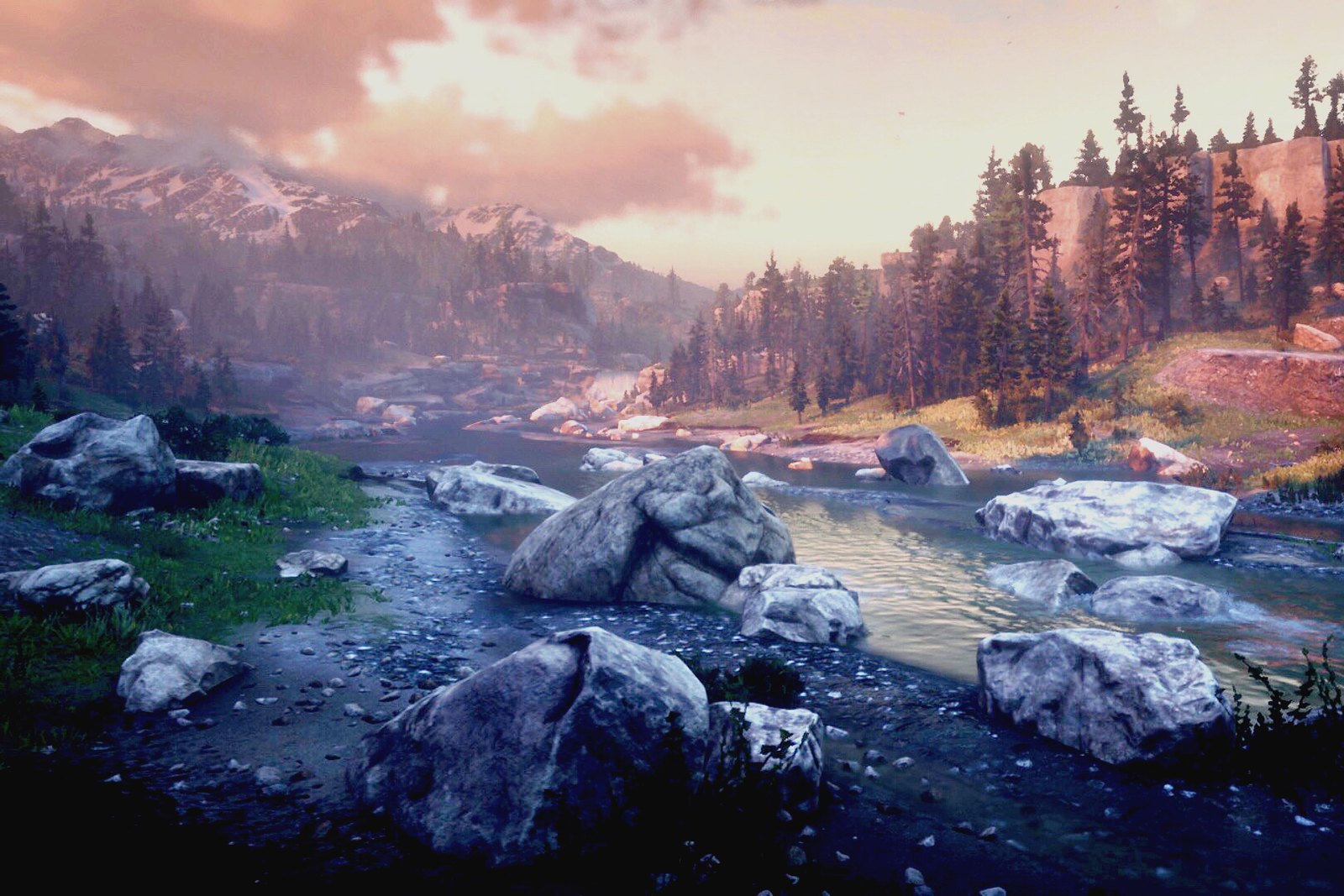This highly detailed and vivid game screenshot depicts an immersive in-game landscape with modern graphics. The scene showcases a serene yet dynamic environment featuring a small creek or river, which originates from the base of a distant, snow-capped mountain visible in the top left corner. This mountain is shrouded by grey clouds, adding a dramatic touch to the far background.

The river flows to the right, moving out of frame while tracing back to the left where it begins at the mountain base. The surroundings of the creek display a blend of natural elements; large stones are scattered across a muddy or dirty patch along the riverside. Adjacent to this patch on the left, a verdant grass area with additional rocks provides contrast to the muddy terrain. 

On the opposite side of the river, the landscape transitions to a sunnier, brighter scene, featuring lush grass and a dense array of pine trees standing before a rugged stone hillside. The lighting on this side enriches the vibrant greenery, creating a visually striking panorama.

In the foreground, behind one of the stones by the creek's left bank, a crouching man with a tattered shirt and frizzy hair can be seen partially obscured in the shadows. His back is to the camera, placing the viewer in a typical third-person perspective common in video games, enhancing the immersive experience. The identity of the figure remains enigmatic, adding an element of mystery to the captivating landscape.